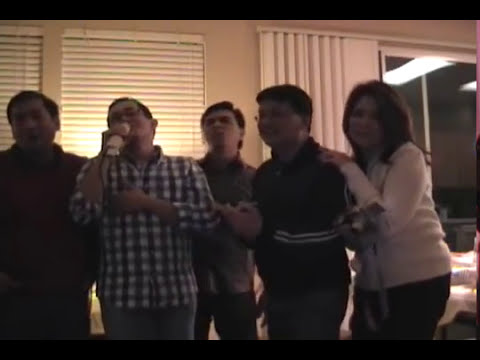The image captures a lively moment inside a room featuring a group of five adults, standing in front of a white wall adorned with two windows on the left and a large window on the right, all dressed with white blinds and curtain, respectively. The room appears dimly lit, enhancing the cozy atmosphere likely reminiscent of an old camcorder recording. In the foreground, three men on the left are deeply engaged in singing, with the second man from the left passionately holding a microphone in his left hand against his chest and donning a white and blue plaid shirt paired with jeans. The men surrounding him also appear animated, contributing to the joyous scene with their open mouths, singing along. Completing the group, a fourth man stands beside them in a black Adidas jacket, distinguishable by its white stripes. On the far right, a woman with long brown hair and light skin stands wearing a white shirt and black pants, gently resting her hand on the shoulder of the man beside her, adding a touch of camaraderie. The overall scene is cropped by thin black strips at the top and bottom, emphasizing the nostalgic charm of this captured moment of friends potentially enjoying a karaoke session.